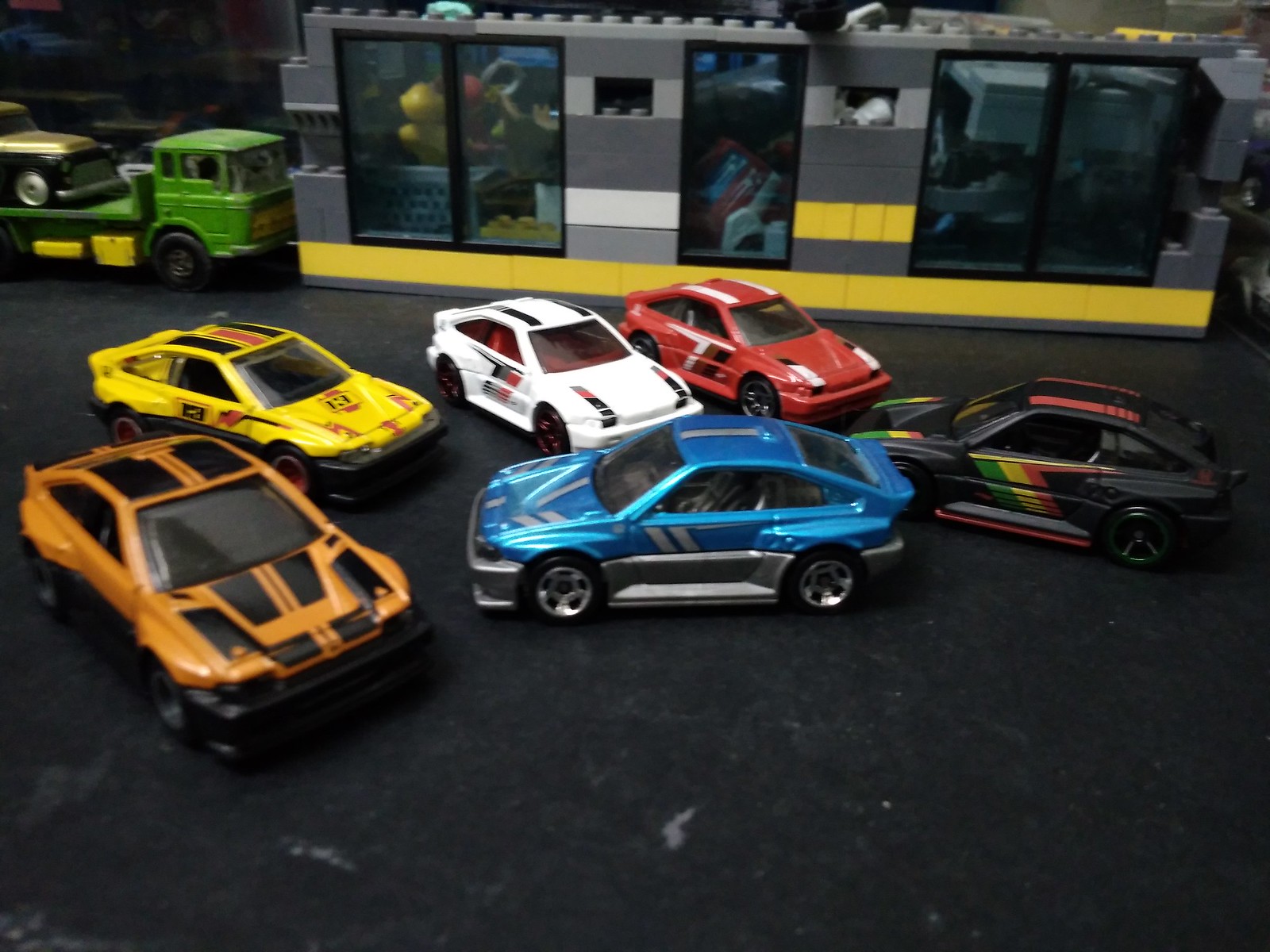The image depicts an assortment of die-cast toy cars arranged on a black surface. Prominently featured are six vibrantly colored cars: an orange car with black stripes resembling a Maserati, a blue car with gray accents similar to a Mustang, a yellow car with red accents, a white car with black and red accents and red seats, a red car with white and black accents, and a black car decorated with green, yellow, and red stripes, possibly hinting at a sporty design. In the background, a Lego-built structure, possibly depicting a car lot, a bus stop, or a train station, is visible, featuring small Lego figures. Adjacent to the Lego structure is a green die-cast tow truck carrying a golden car on its flatbed. The Lego building is primarily gray with yellow lines interspersed throughout its design. The scene effectively conveys a playful and intricate setup centered around toy cars and Lego constructions.